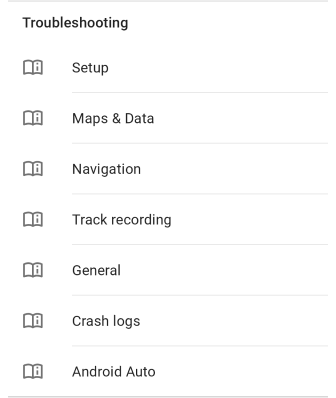The image contains a vertical rectangular box with narrow gray borders on the top and bottom, giving it a framed appearance. Although the sides lack visible borders, the text inside is formatted as if on wide-lined paper. At the top, the word “Troubleshooting” is prominently displayed in a darker font, beginning with a capital 'T' and followed by a white space.

Below this heading, a series of entries are listed, each prefixed by an icon resembling a small book containing an "I" for information. These entries, each separated by a horizontal line, include:

1. **Setup**
2. **Maps and Data**
3. **Navigation**
4. **Track Recording**
5. **General**
6. **Crash Logs**
7. **Android Auto**

This structured format aims to provide users with clear and organized guidance on various troubleshooting topics.